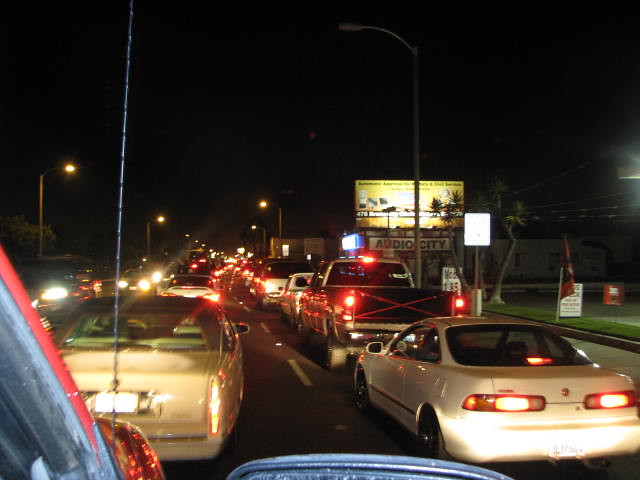This night-time photograph provides a dynamic glimpse of a traffic standstill, captured by someone leaning out of their red car. The image reveals a busy multi-lane road, possibly a highway, with two lanes in each direction. Traffic is at a complete halt, with a multitude of cars, trucks, and vans extending into the distance. On the right side of the frame, a yellow billboard stands out, featuring silhouettes of trees and what appears to be a serene lake with boats. The scene is illuminated by several streetlights against a backdrop of the dark night sky, emphasizing the congestion and the stillness of the moment.